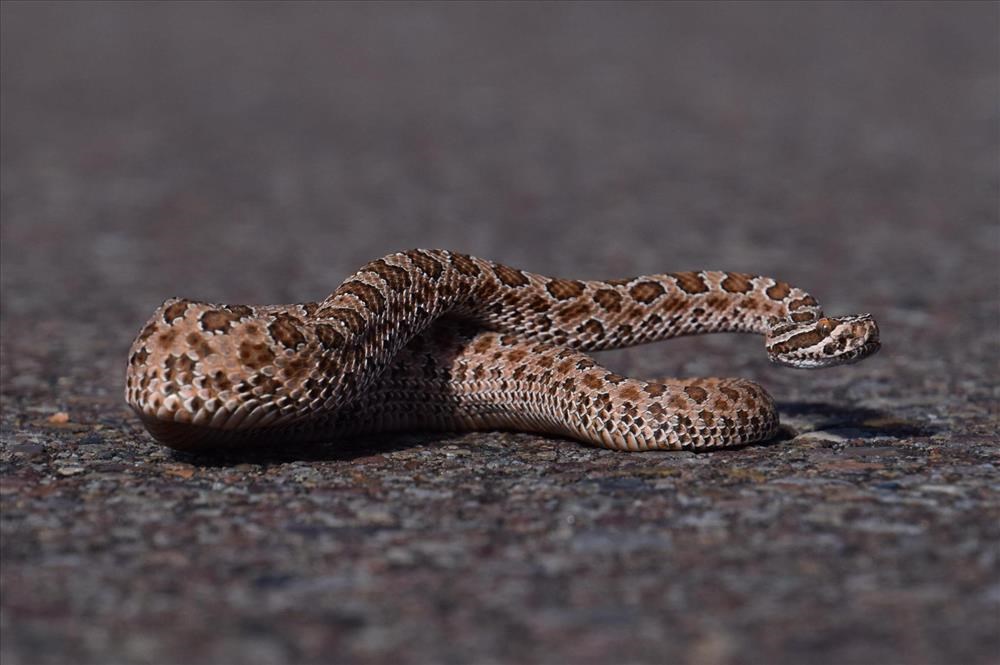The image captures a live snake coiled on a black, roughly textured paved surface, reminiscent of asphalt or stone. The snake, approximately 2-3 feet in length, appears to be in a striking pose with its head raised above the ground. Its body forms a U-shape, partly coiled, making its tail not visible in the photograph. The snake features a tan-brown base color adorned with distinct, orange-brown circular spots outlined in black, along with black diamond patterns running along its back. Its head, small and somewhat tilted upwards, shows no open mouth or visible tongue. The background is deliberately blurred to emphasize the snake, giving the entire scene a bright, outdoor daylight setting. The snake’s physique suggests it has a proportionally thicker middle, possibly indicating a recent meal. The overall appearance hints at the characteristics of a rattlesnake, although the tail and rattle are not visible.